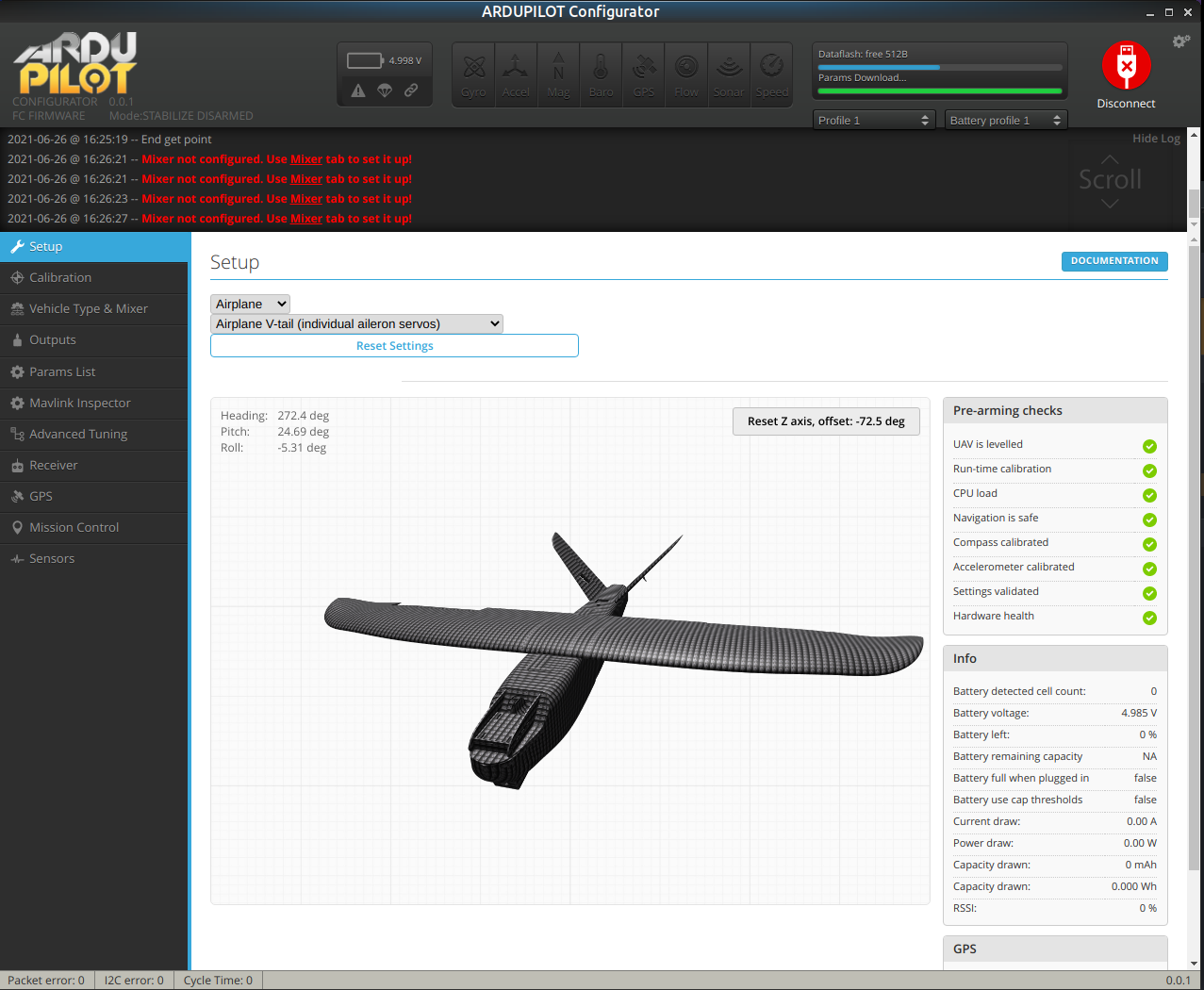The image is a detailed screenshot of the ArduPilot Configurator interface on a computer webpage. At the top, a blue banner displays "ArduPilot Configurator" in white text, along with standard window control buttons – an 'X' for closing, a minimize button, and a maximize button. The ArduPilot logo, featuring white and yellow colors, is prominently placed next to the text "Configurator 0.01 FC Firmware."

To the right of the interface, a graph is visible. A blue bar above the graph reads "DataFlash Free 512B," and the "Params download" status is indicated in green. A prominent red "Disconnect" button signifies the option to disconnect the USB connection. 

On the left side of the interface, a black vertical banner lists various tabs: Setup, Collaboration, Vehicle Type and Mixer, Outputs, Params, List, MAVLink, Inspector, Advanced Tuning, Receiver, GPS, Mission Controls, and Sensors. The "Setup" tab has been selected, revealing its contents in the main view.

Central to this view is a detailed simulation of a small aircraft, showcasing the virtual model and settings linked to the setup tab.